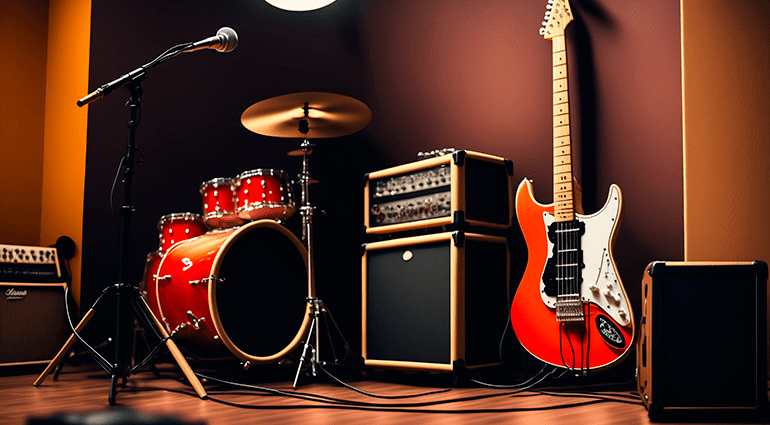The image depicts an AI-rendered music studio setup with various instruments poised for a performance. The scene captures a horizontal view in a dark studio environment with walls of burnt orange and deep purple tones. Dominating the center, there's a tall amplifier stack filled with numerous knobs and dials and a speaker at the bottom. To its right stands an electric guitar on a stand, featuring a red body, black fretboard, and white background, with a light brown wooden neck and a black oval shape near the headstock's tuning pegs. Beside the guitar, another speaker rests on the floor. 

To the left of the amplifier stack lies a vibrant drum set, consisting of one large bass drum and three smaller drums above it, all accented by a stand-mounted cymbal. The drum set shows an array of colors, mainly red with an orange bass drum and silver hardware. At the far left of the image, a microphone stand, angled at the top, stands near the drum set. Additionally, there is another amplifier stack faintly visible in the corner at the far left side of the frame. The stage exudes a beautiful wooden texture, enhancing the rich, colorful ambiance of the studio.